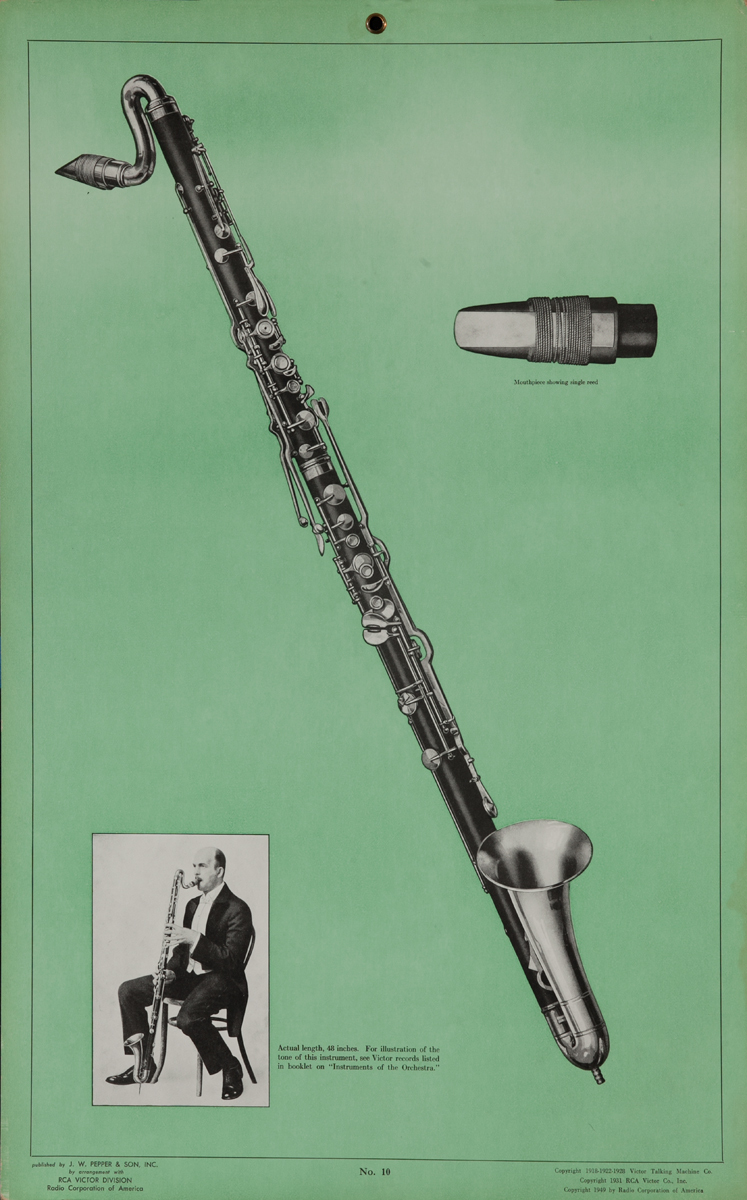This image appears to be an old advertisement for a long, metal musical instrument, most likely a woodwind, possibly a clarinet or a type of oboe. The instrument is depicted lying against a dull green background bordered by a black line. The top right of the image contains a close-up view of the intricately shaped, curved mouthpiece. The instrument itself is quite long and slender with many buttons along its body, which is predominantly black in the black-and-white image.

In the bottom left of the poster, there is a smaller inset showing a man seated on a chair, playing the instrument. The bottom part of the instrument touches the floor while the top part reaches up to his mouth. This inset further confirms the instrument's length and form, ending in a flared bell similar to that of a clarinet but narrower than a trumpet. The overall appearance and design elements suggest it is from the woodwind family.

Surrounding the image are various blocks of black text, particularly below the close-up of the mouthpiece and around the top, right, and bottom edges of the poster. However, the text is too small and indistinct to make out clearly. The vintage and somewhat degraded quality of the image enhances its old advertisement aesthetic. The poster seems to aim at showcasing or advertising an old, likely historical, woodwind instrument.